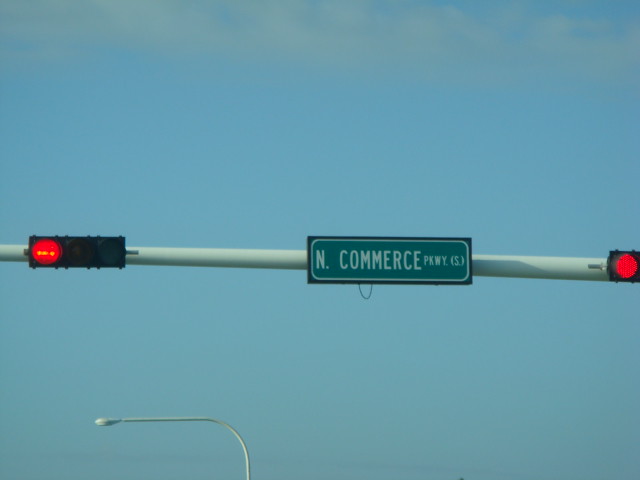This daytime photograph captures a vibrant street scene featuring a street sign mounted on a horizontal, white, light gray metal stoplight pole. The pole supports two red traffic lights, positioned flush against it. In the center of the pole, a green street sign with white text prominently displays “N.COMMERCE” in large font and “PKWY.S” in smaller font within parentheses, indicating North Commerce Parkway South. The photo showcases a clear blue sky dotted with white fluffy clouds, which grow slightly grayer towards the horizon. A white streetlight protrudes at a 90-degree angle from the lamppost in the background. Shadows suggest the primary light source is above and behind the camera. The ground is not visible in the shot, emphasizing the sky, sign, and traffic lights.